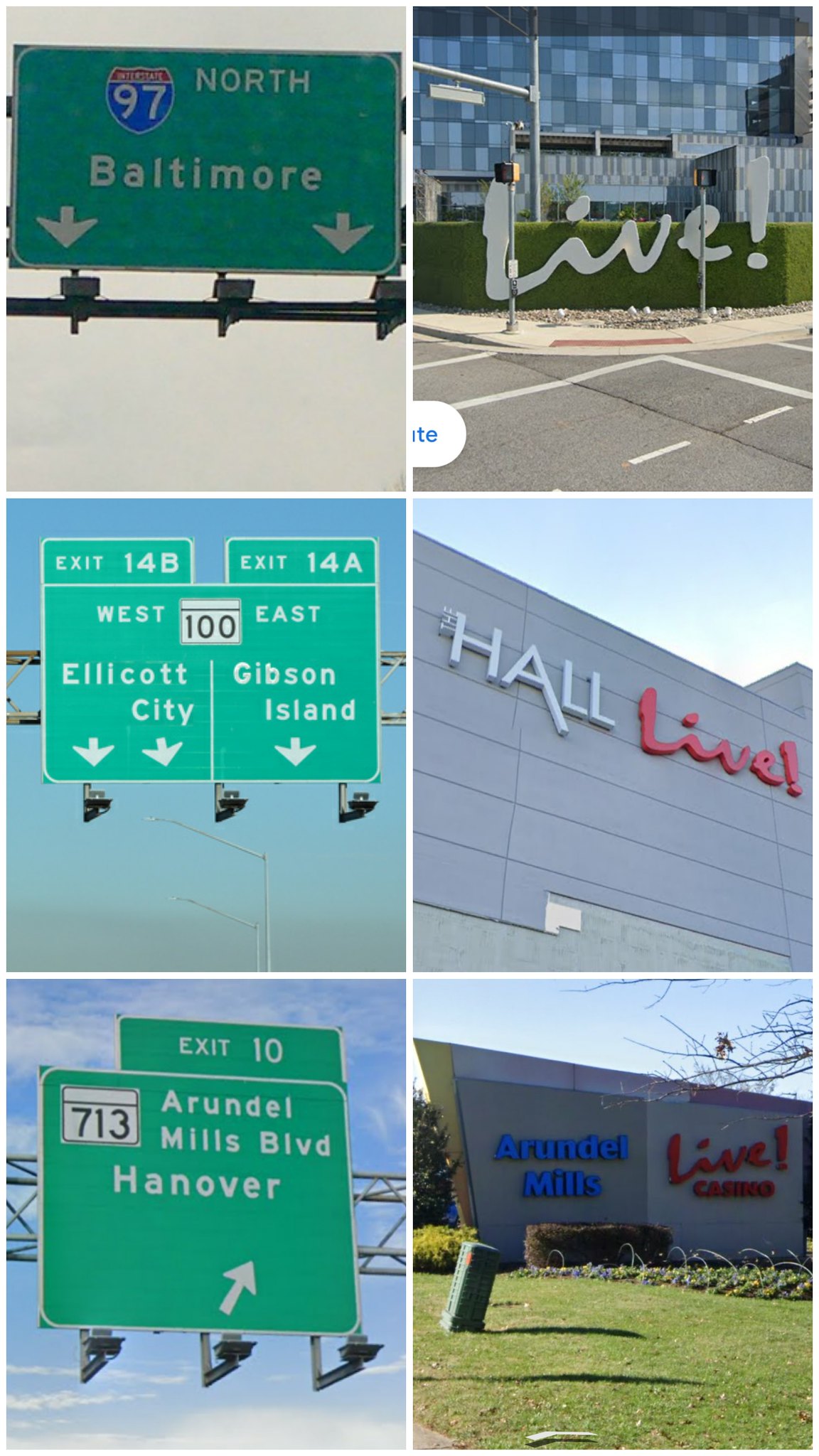This collection features six captured images of street and store signs, displayed in a grid separated by white lines. 

- **Top Left Corner:**
  - **Image 1:** A green interstate highway sign displaying the Interstate 37 emblem with the text "North". Below that, it reads "Baltimore" and includes two downward-pointing arrows.
  
- **Top Center:**
  - **Image 2:** An intersection scene with a sign placed against a bush that reads "Live!" in bold text.
  
- **Top Right Corner:**
  - **Image 3:** A highway sign indicating "Exit 14B" and "Exit 14A", with directional labels beneath, reading "West" and "East". "Elliott City" is listed on the left side and "Gibson Island" on the right, each with down-pointing arrows.

- **Bottom Left Corner:**
  - **Image 4:** A building sign with vibrant red and yellow text reading "Hall Live".
  
- **Bottom Center:**
  - **Image 5:** Another highway exit sign that says "Exit 10, 713, Arundel Mills Boulevard, Hanover" with an arrow pointing to the upper left.

- **Bottom Right Corner:**
  - **Image 6:** A sign marked "Arundel Mills" featuring the word "Live" prominently.

Each image presents a distinct street or building sign, contributing to a diverse and vivid portrayal of urban signage.